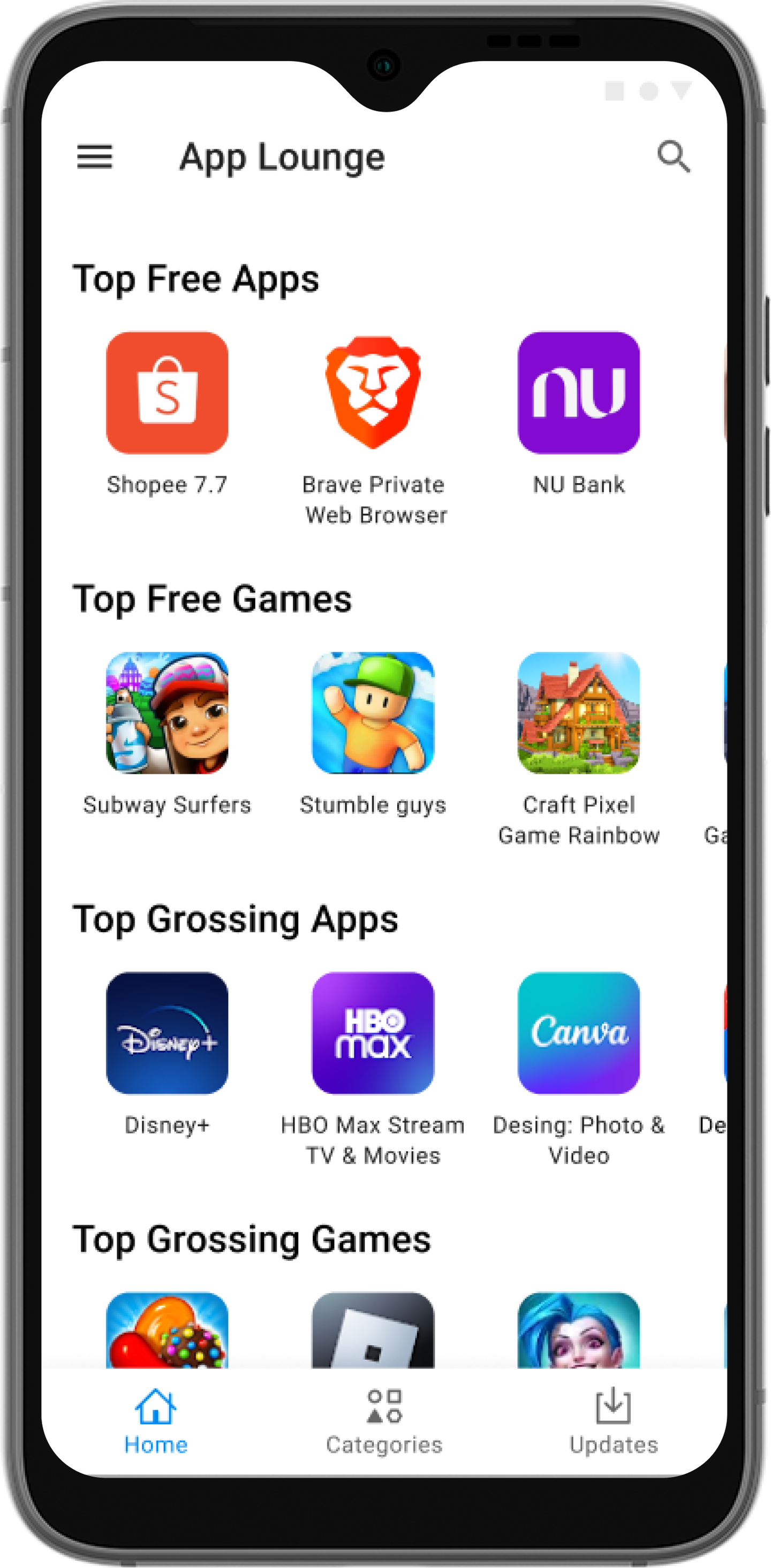A sleek, black phone with silver edges is depicted in this image. The screen showcases a variety of apps and elements in meticulous detail. Towards the top right of the screen, there's a hamburger icon and an apple with ham, arranged in a square, circle, and triangle. Below this, the top three apps are displayed: a square shopping bag labeled "Essence," the "Shoppy 7.7" app, and a private web browser. A line connects to an app called "Nubix," which is represented by a purple square icon.

Further down, the top three games are listed: "Subway Surfers," featuring a character with a baseball cap and a spray can; "Tumbleguys," showing a character with a green cap, orange shirt, blue pants, against a blue sky with white clouds; and "Rooftop Craft Pixel Game," illustrated with a rainbow. Among the top grocery apps, the icons for Disney+ and HBO Max are visible, with HBO Max highlighted in purple. 

In the TV and movies combo section, there's a reference to a train and photo and video content. The top grossing games include "Candy Crush," represented by a colorful square containing a cube, and an icon of Jinx from "League of Legends," who is smiling. The image also features a gingerbread figure, poised to be eaten.